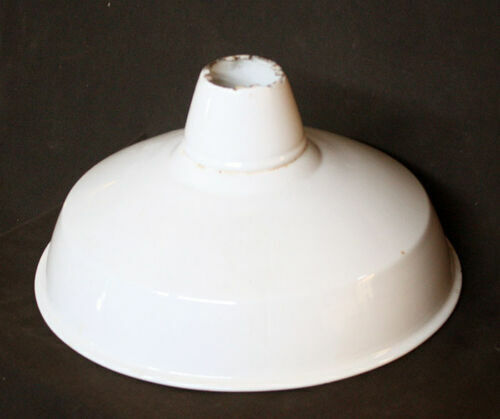The image depicts an intriguing white object set against a stark black background, creating a striking contrast. This object, which appears to be metallic and slightly shiny, is notably whiter at its base and features a small lip at its end. The shape resembles an upside-down lamp or possibly a funnel-like structure, with a round, wide base that tapers into a narrower, rough-edged top, suggesting it might have been cut or broken off. The surface around the opening at the top appears to be slightly dirty. The object's precise purpose is unclear, but its clean lines and utilitarian design suggest it might be some kind of functional item. The absence of any other objects or background details makes it difficult to determine the object's scale or specific use.